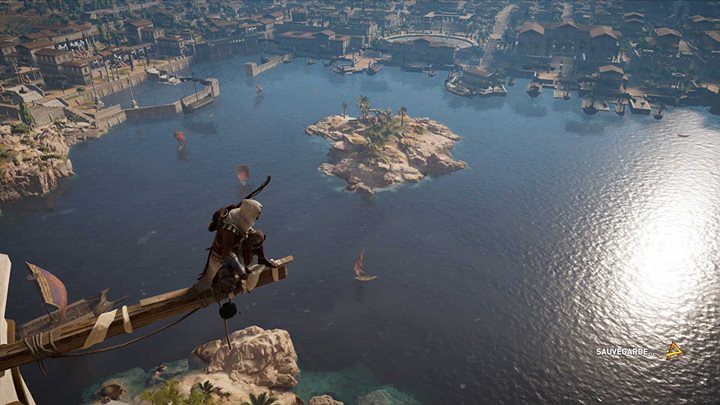This captivating image appears almost surreal, resembling a scene from a video game or a digitally-generated creation. Dominating the left side of the picture is a wooden pole jutting out seemingly from nowhere. Perched at the far end of this pole is a figure, who appears to be surveying the scene below. This person wears a white cloth draped over their head, and bears a bow and arrow slung across their back. They are either shirtless or clad in a reddish-brown top, paired with a white, skirt-like garment and sturdy boots, giving them an enigmatic, almost mythical appearance.

Directly beneath this figure, jagged rocks emerge from the steep cliff which plunges into the dark, deep ocean. The water, a mesmerizing blend of turquoise near its meeting point with the shore, contrasts starkly with the silhouettes of distant city structures. The sprawling city in the background features predominantly brown buildings with reddish roofs, yet it exudes an eerie, abandoned atmosphere due to the absence of visible inhabitants.

Interspersed among the city's architectural expanse is a small rocky island adorned with palm trees, adding a touch of tropical flair. Amidst the waves below, a lone surfer is seen riding the water, providing the sole hint of active life in this otherwise desolate townscape. The ocean itself occupies a significant portion of the image, enhancing the sense of solitude and mystery.

In the lower right corner of the image, the word "Sauvegarde" is elegantly inscribed in gold, accompanied by a small, intricate symbol. This label adds a final touch of intrigue to the scene, leaving viewers to ponder its meaning and the story behind this vivid tableau.